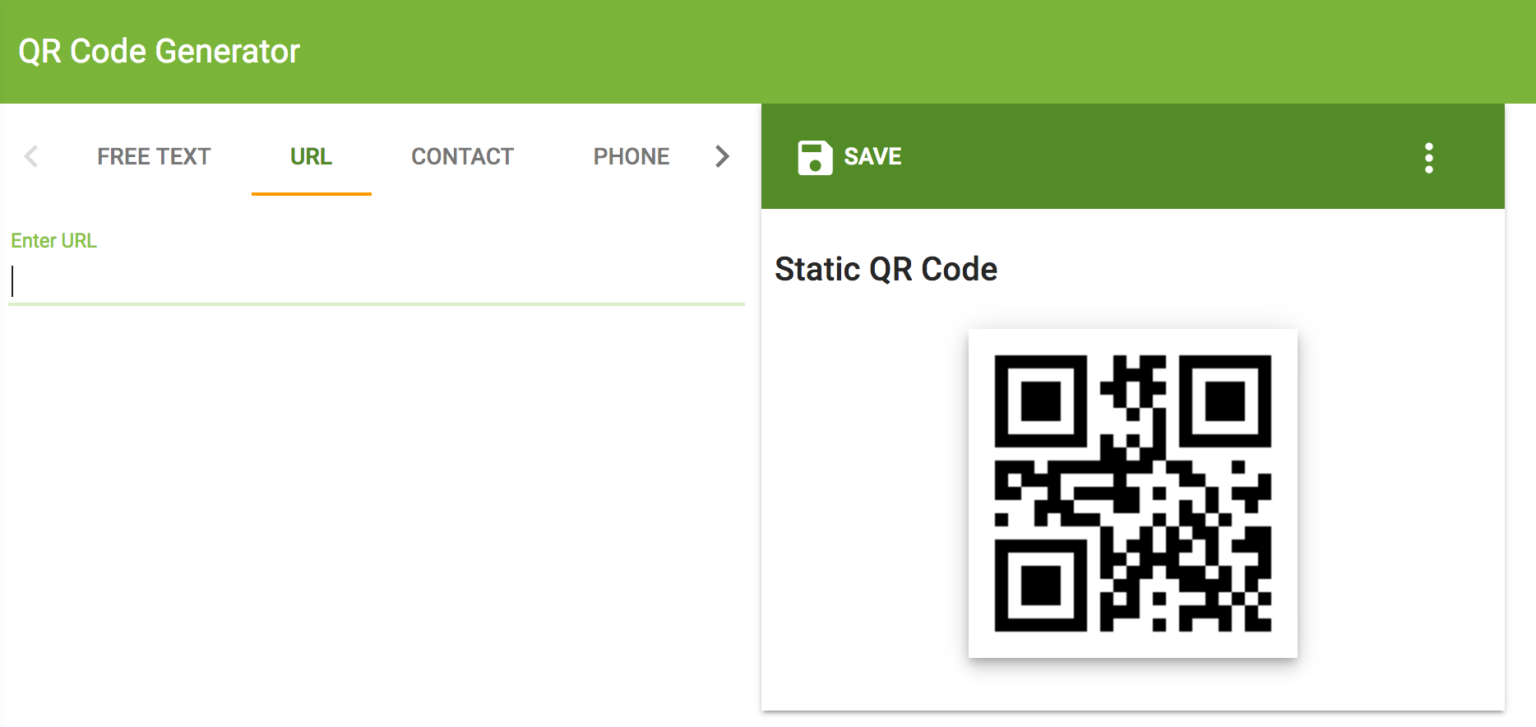The image predominantly features a user interface for a QR code generator. The background is a mix of green, white, and black elements. At the top, a green bar spans the width of the image, with the words "QR Code Generator" in white text positioned in the upper left corner. Below that, there's a horizontal white rectangle containing clickable options labeled "Free Text," "URL," "Contact," and "Phone" in black text, with "URL" highlighted by an orange underline indicating its current selection.

Under the rectangle, a text box labeled "Enter URL" is visible, suggesting that users can input a URL here. Adjacent to this text box on the right, there is a darker green bar with a white "Save" button, accompanied by a small symbol just to its left. To the right of this green bar, there are three vertical dots, indicative of a menu option that can be expanded for additional features.

Beneath these elements, the interface displays a larger white rectangular box. At the top of this box, black text reads "Static QR Code." Below this text, within the white rectangle, there is a black and white static QR code that users can presumably scan. Overall, the image portrays a detailed and functional QR code generator interface.